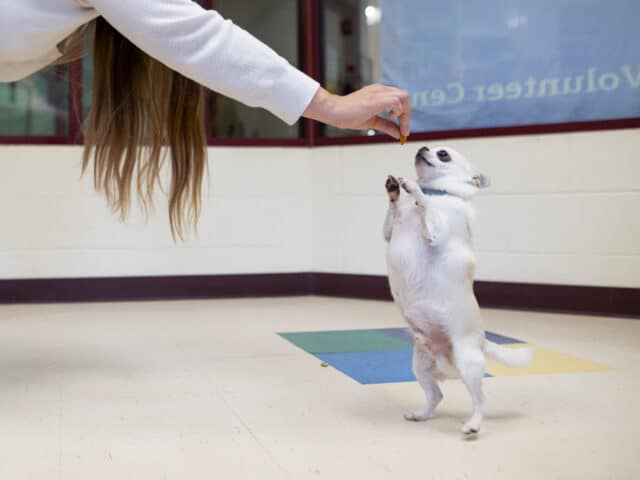The photograph features a small, white Chihuahua standing on its hind legs, likely undergoing training or performing a trick. The dog, which appears to be somewhat overweight and muscular at the top, is reaching out for a treat held by a woman. The woman’s long brown hair with blonde highlights can be seen trailing into the picture. She is wearing a white long-sleeved shirt, although another description suggests she has on a red sweater. The dog, identifiable by its big black eyes and distinct black or brown markings around them, is wearing a blue collar. In the background, there are large windows and white concrete brick walls, which indicate that the setting might be a veterinarian or volunteer center, as suggested by the partially visible letters "V O L U N T E E R C E N" on the wall. The floor is primarily cream-colored with a square pattern incorporating green, yellow, blue, and purple squares.